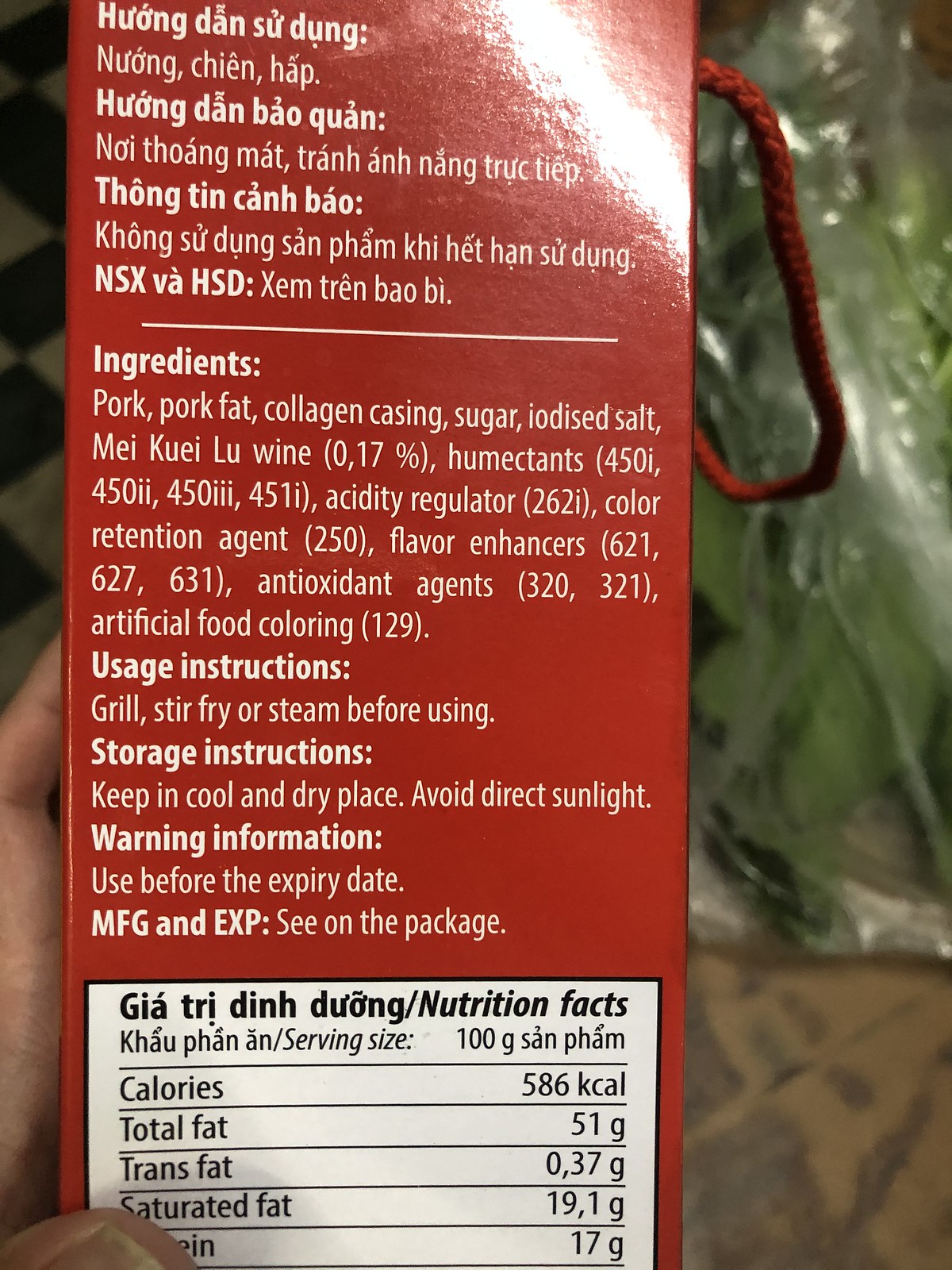The image depicts a shiny red cardboard package of food that is being held by a person's hand on the left side, with their thumbnail visible in the lower left corner. The package features a woven handle possibly indicating it's placed above a kitchen floor or prep space. The text on the box includes both Vietnamese, recognizable by its accented characters, and English. The visible sections showcase the ingredients list stating pork, pork fat, collagen, casing, sugar, and iodized salt, suggesting it contains a meat product, likely sausage or another cookable meat item. Detailed instructions specify that it should be grilled, stir-fried, or steamed before consumption. Storage guidelines advise keeping it in a cool, dry place, away from direct sunlight, and to use it before the expiration date. The nutrition facts reveal the product has 586 calories and 51 grams of fat, indicating a high-fat content.